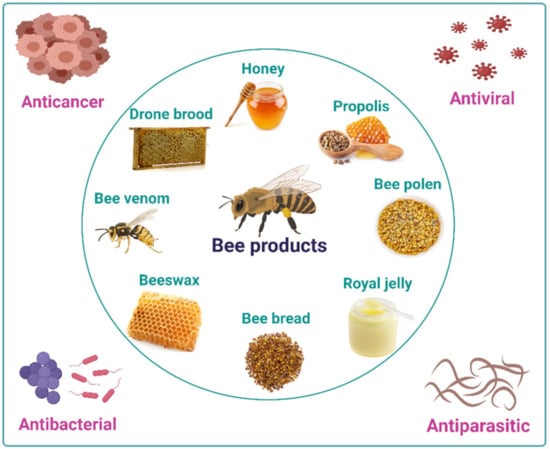This detailed infographic showcases the benefits of various bee products within a white square trimmed with a turquoise blue border. Central to the design is a blue-outlined circle, featuring a large bee in the middle with the text "Bee Products" prominently displayed below it. Surrounding the bee, the circle contains images and labels of different bee products arranged in a clockwise manner: starting at 12 o'clock with honey, followed by propolis, bee pollen, royal jelly, bee bread, beeswax, bee venom, and finally drone brood around 10-11 o'clock. Each product name is written in green, and a corresponding image is provided.

In each corner of the infographic, there are thematic illustrations with labels written in purple, highlighting different health benefits of bee products: 
- The top right corner displays "Anti-Cancer," accompanied by an image that resembles pink overlapping circles, possibly flowers or honeycomb.
- The top left corner indicates "Anti-Viral," represented with an image of flowers.
- The bottom left corner is labeled "Anti-Bacterial," featuring images of grapes and bacteria.
- The bottom right corner reads "Anti-Parasitic," illustrated with swirling motifs.

The combination of vibrant images, health benefit labels, and detailed arrangement offers an informative and visually engaging summary of the diverse advantages provided by bee products.